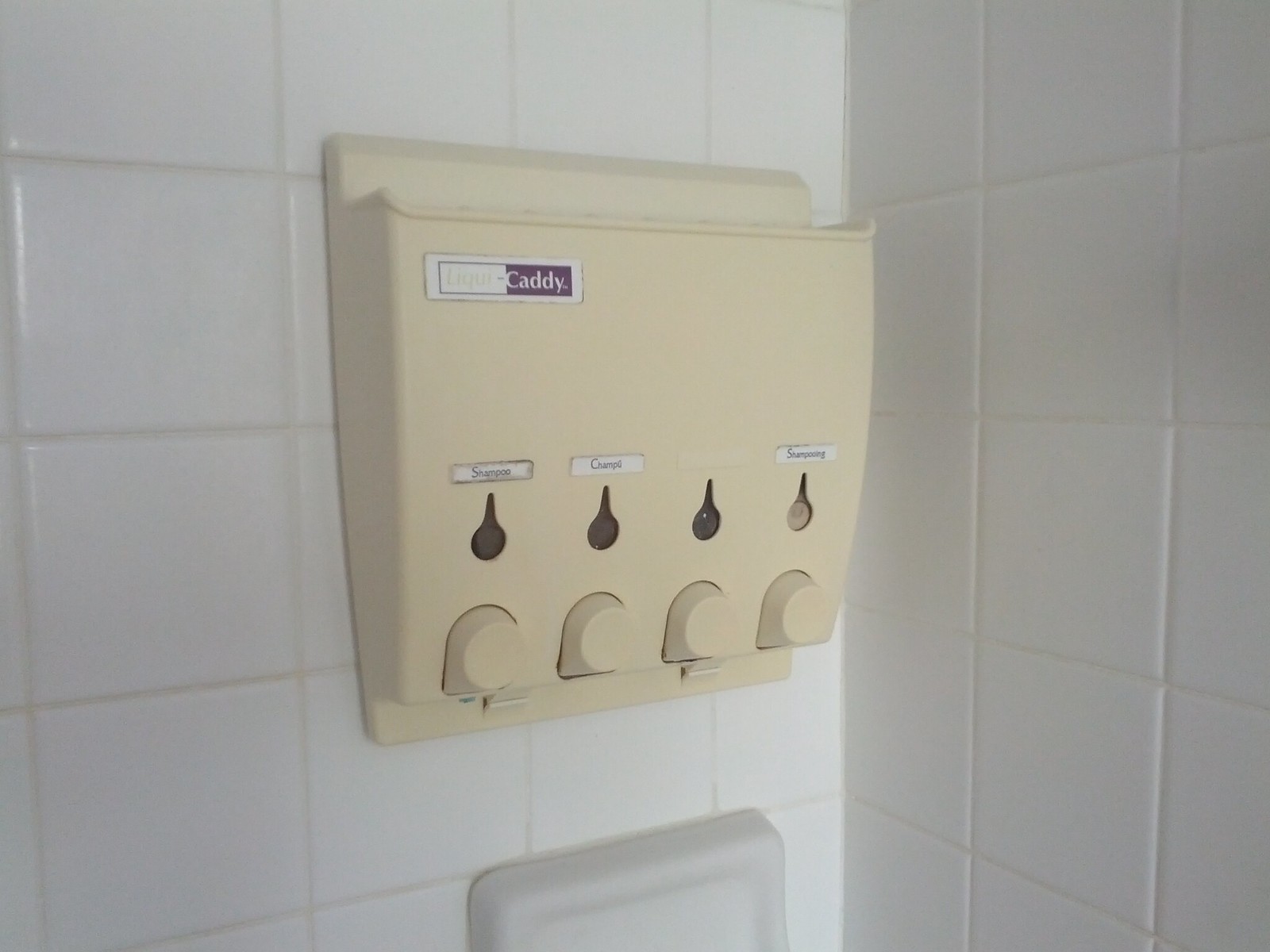The image depicts a detailed view of a shower corner with white tile walls, partially showing both the right and left sides. Prominently featured up against the left-hand wall is a plastic, light tan shower caddy. This rectangular caddy adheres to the wall, with an open-top shelf designed to hold items. Positioned at the top left corner of the caddy is a two-tone logo, split into white and brown halves, with "Caddy" inscribed in white letters. Below the logo, the caddy displays a series of three teardrop-shaped, brown spots aligned horizontally, each accompanied by small, unreadable labels above them. Further down, under each teardrop shape, are dome-shaped dispenser outlets, likely used for dispensing shampoo or other toiletries. At the very bottom of the image, beneath the caddy, part of a white porcelain soap dish is visible, blending into the tiled backdrop.